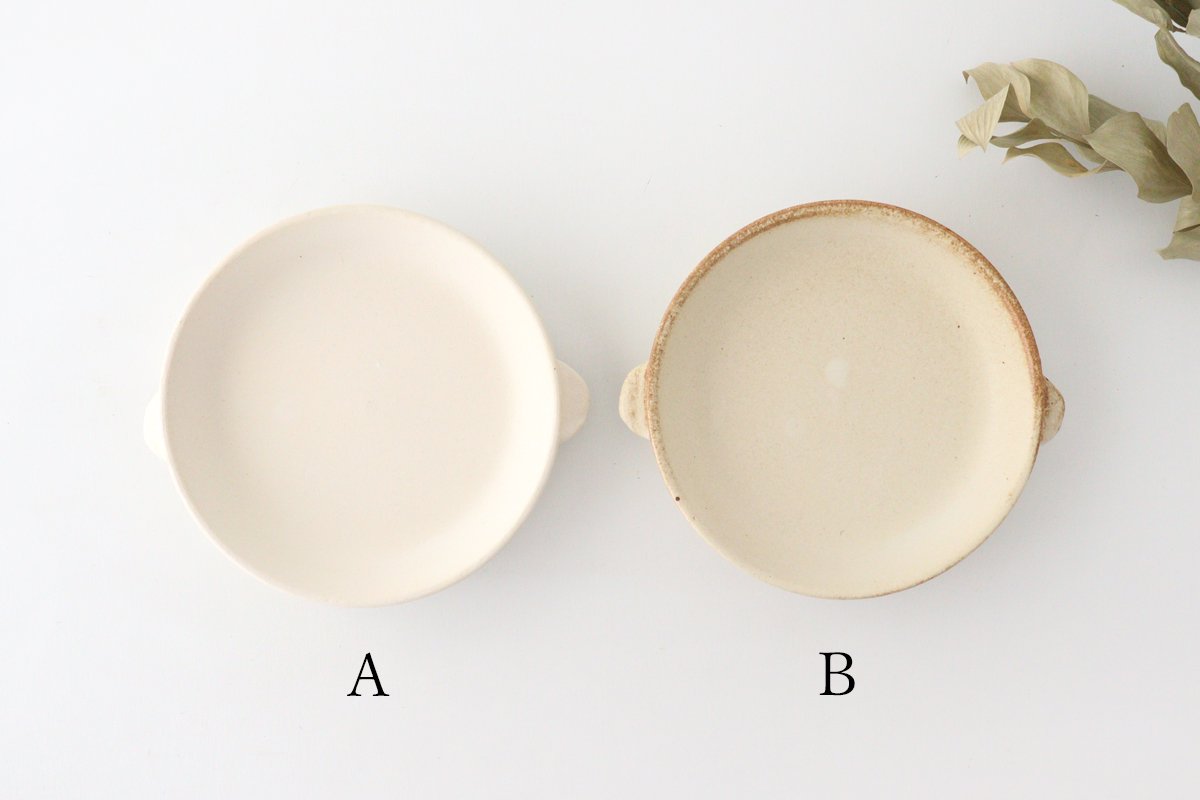In the image, we see two bowls viewed from above, each occupying the left (labeled A) and right/middle (labeled B) sections of the frame. Bowl A is a pristine white porcelain dish with two handles, one on each side. In contrast, Bowl B, which appears to be older, is slightly darker with beige tones and a distinct brown outline around the rim. This bowl also features similar handles but bears marks of usage, with some brown markings present. Both bowls are empty and rest on a white background that is brighter on the left side. In the upper right corner of the image, there is a sprig of dried vegetation, possibly bay leaves, adding a subtle natural element to the composition.